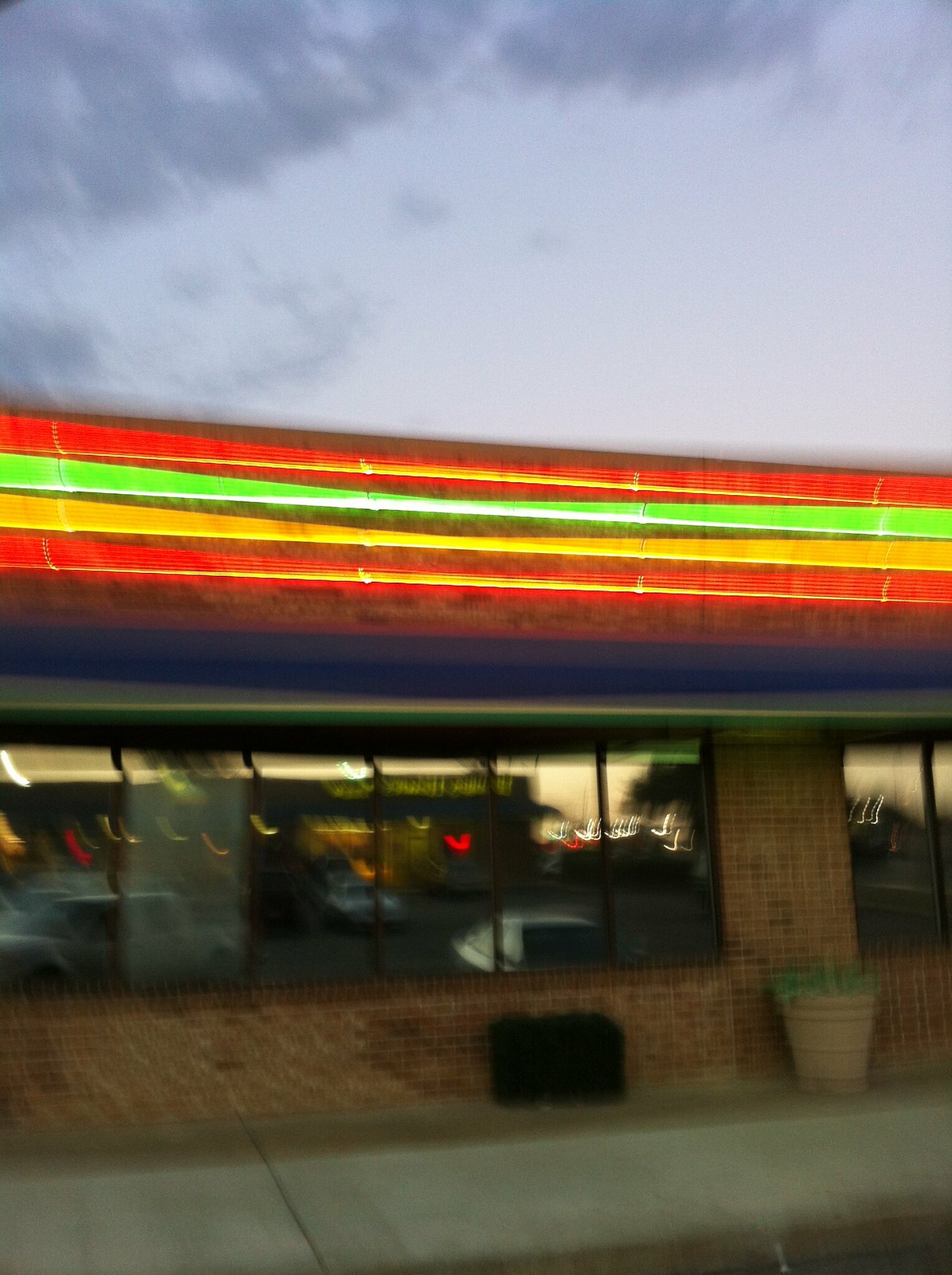This vertical, slightly blurred image captures the exterior of a red-brick restaurant from the cement sidewalk in the foreground to the sky above its flat roof. The sky exhibits a rich, darkening blue hue adorned with ominous cumulonimbus clouds. The roof of the restaurant features vibrant neon bands—encased in a protective plastic covering—stretching from top to bottom in sequences of red, green, yellow, and red. Below these neon accents is a black base, possibly an awning or structural foundation for the roof. The restaurant itself boasts large, multi-paned windows that mirror the surrounding buildings, providing a dynamic, reflective glimpse into the adjacent area.